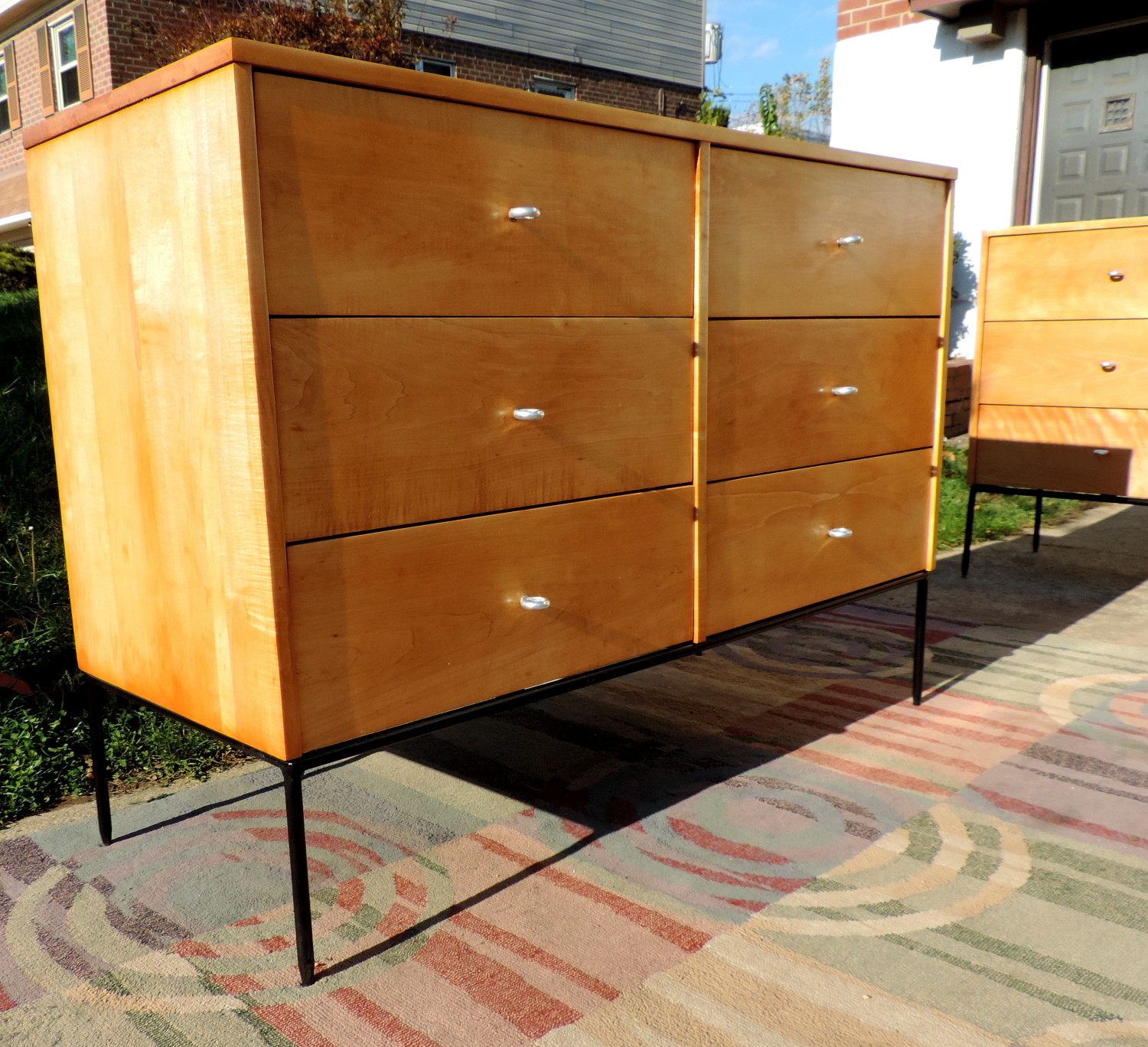The photograph captures an outdoor scene featuring two nearly identical wooden dressers. The primary dresser dominates the frame, showcasing its simple design with pale, oaky wood and wide drawers arranged in three rows and two columns. Each drawer has a small metal handle at its center. Behind it, the blue sky peeks through, framing a white house with a black door. Below, the dressers appear to rest on a patterned carpet laid over a cement deck. The carpet's intricate geometric designs add a dash of color with stripes in red, pink, tan, green, and black. Both dressers seem to stand on thin black metal legs, or they might be mounted on black coffee tables with metal bars. The secondary dresser, partially visible, mirrors the design of the primary one but only shows one column of drawers. The sun, likely morning light, casts gentle shadows from the left, suggesting the early part of the day.